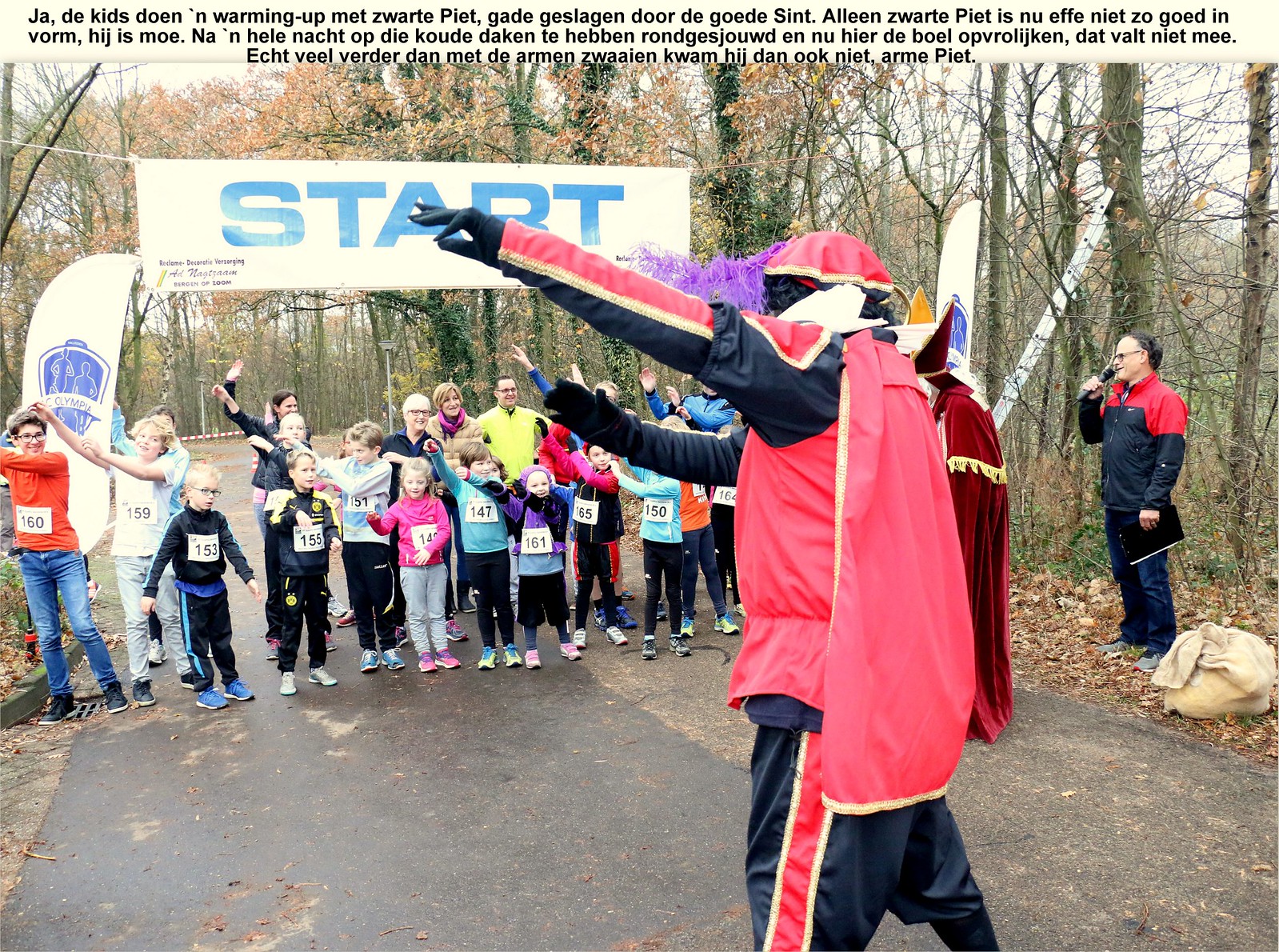In the image, a race is about to begin at a start line marked by a large rectangular banner with "START" written in blue uppercase letters on a white background. The scene takes place on a pavement surrounded by leafless or partially brown-leaved deciduous trees, indicating it might be winter. At the forefront stands a figure dressed in a red and black attire, resembling a harlequin or a performer, complete with a red cape, black pants, a red hat, and a black sleeved shirt. This individual is pointing to the left, and the crowd behind him, consisting of both children and adults, are mimicking his gesture. The children, appearing to be between the ages of 5 and 12, and their likely parents, are all wearing various racing numbers and bibs. At the right side of the image, another person, possibly an event organizer, is holding a microphone. Above the scene, there are several lines of text in what seems to be German, further detailing the event.